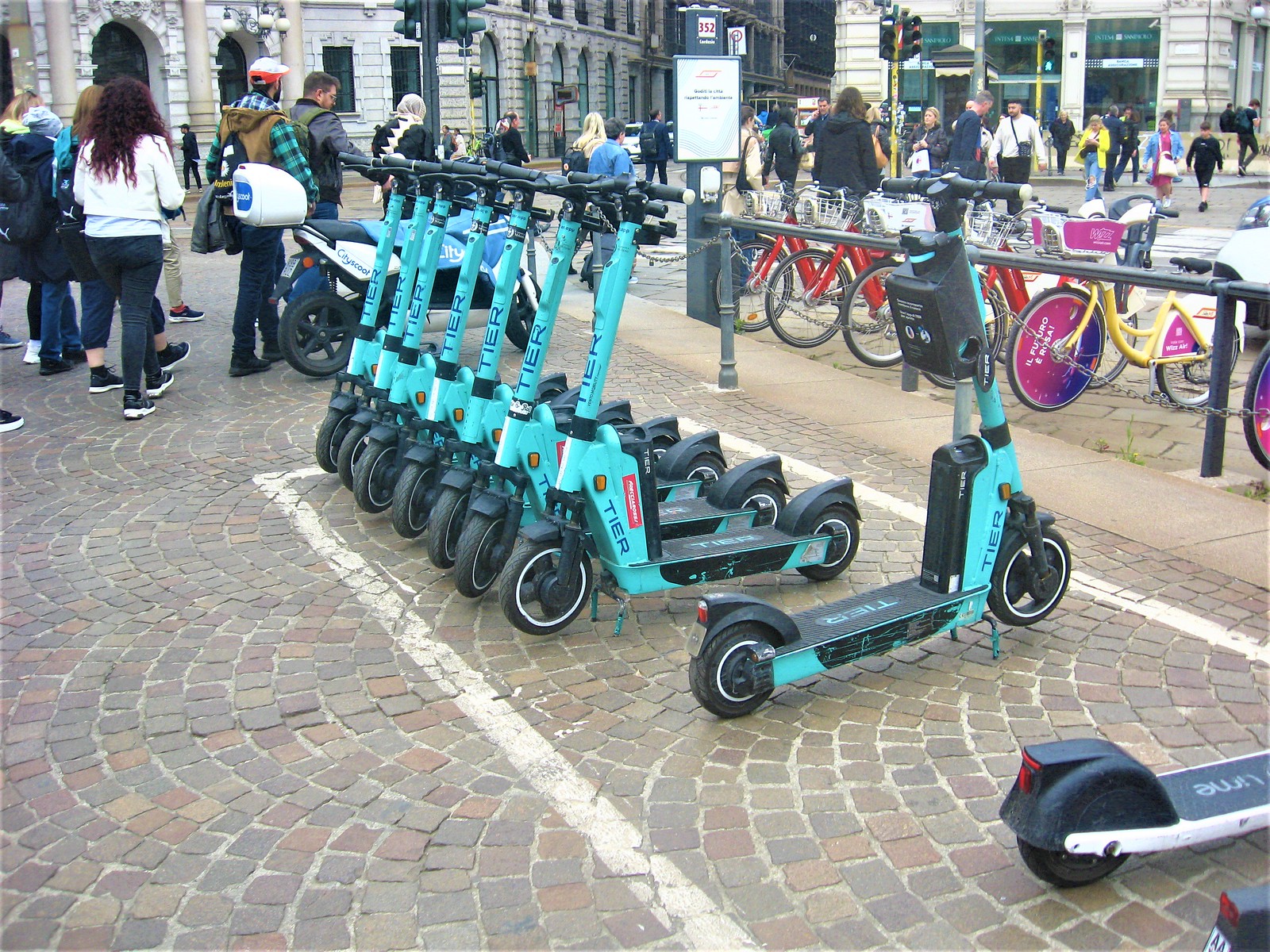In this bustling town square, vibrant with activity, the photograph captures an expansive view of a cobblestone ground in rich, varied hues of reddish-brown, gray, and purplish-red. The central focus reveals several baby blue, motorized scooters, neatly aligned within a white painted rectangle, demarcated on the cobblestones. The scooters, made to resemble traditional kick scooters but with a motorized twist, predominantly face towards the left and are chained together in rows that occupy most of the foreground's left side. However, the lower right corner of the image shows only a couple of scooters, revealing some empty spaces.

To the back and extending into the upper left, a diverse crowd of people traverse the street, encapsulating the lively atmosphere. In the background, majestic, old architectural buildings rise, showcasing their tan and white facades with large arches, intricate ridged textures, and ornate pillars stretching up their exteriors. These buildings frame the scene and offer a glimpse into the historical elegance of the area.

Just to the right of the scooters, a metal fence runs parallel to the street, adorned with various bicycles. Notably, there are several red bikes with silver baskets, and a striking yellow bicycle detailed with black tires and purple-pink accents. Partially obscured by a chain, the lettering on this bicycle suggests it's marked in a non-English language. Further enriching the scene, people walk across the street behind these bikes, moving between black poles that segment the space. Ensuring safety and order amidst the hustle, traffic lights rise along the street, their signals partially visible in the photo.

This detailed snapshot encapsulates a harmonious blend of modern mobility, historical splendor, and the ceaseless ebb and flow of urban life.